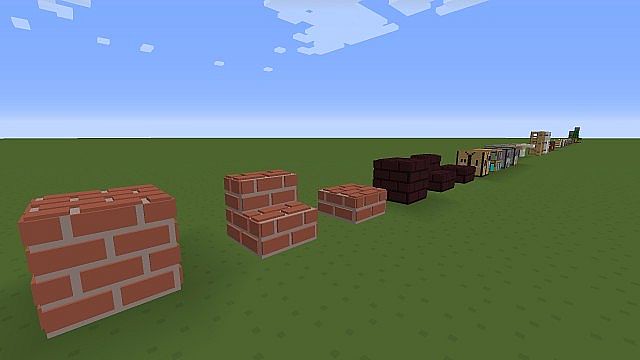This rendered image depicts a pixelated field of grass under a light blue sky, adorned with off-white, block-shaped clouds reminiscent of Minecraft or Roblox aesthetics. A series of blocky objects stretches diagonally from the bottom left corner to the horizon across the green terrain. These objects primarily consist of brown bricks with light-colored masonry and appear to be constructed from large square blocks. Intermixed with these are black squares, some featuring green, blue, or turquoise hues. The overall color palette from the camera's perspective is dominated by shades of brown, off-white, and black, creating a visually striking yet minimalist scene.